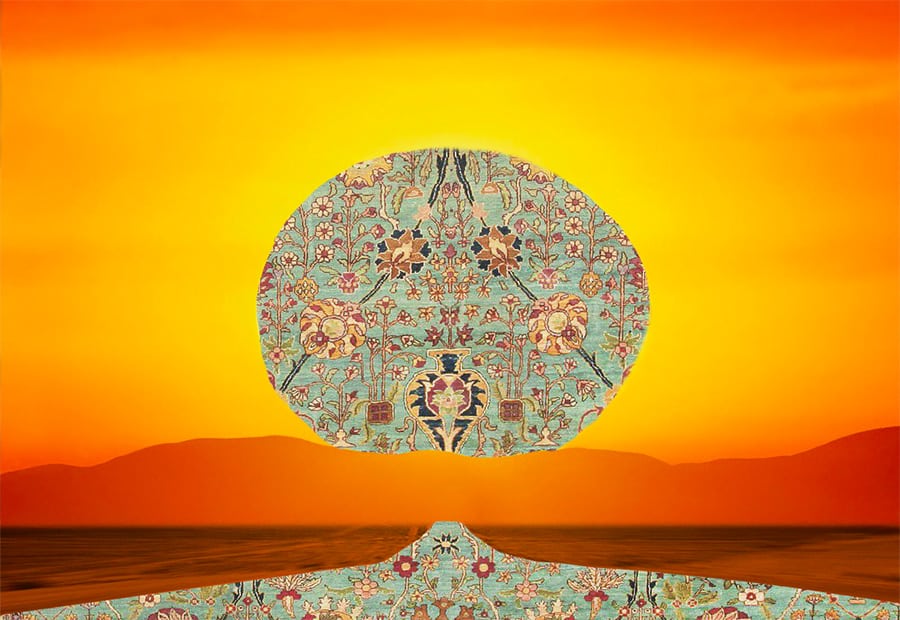This image depicts an abstract scene dominated by vibrant colors and floral motifs. At the center, a round-shaped element adorned with oriental flowers, daisies, and a vase brimming with flowers fades into the distance. The round shape showcases a spectrum of colors including orange, red, yellow, green, and blue, set against a light blue background. A path, composed of multi-colored flowers and leaves, winds from the left to the right, narrowing as it converges towards the bottom center of the image. Flanking this floral path are desolate orange areas reminiscent of sand dunes. On the horizon, an orange mountain range can be seen beneath a sky bathed in shades of yellow and orange, evoking the hues of a sunset. Above the mountains, a surreal sun crafted from the same blue floral pattern as the path adds to the fantastical atmosphere. The overall color scheme transitions from deep oranges at the top to lighter yellows closer to the path, creating a cohesive and warm scene that merges natural elements with imaginative artistry.